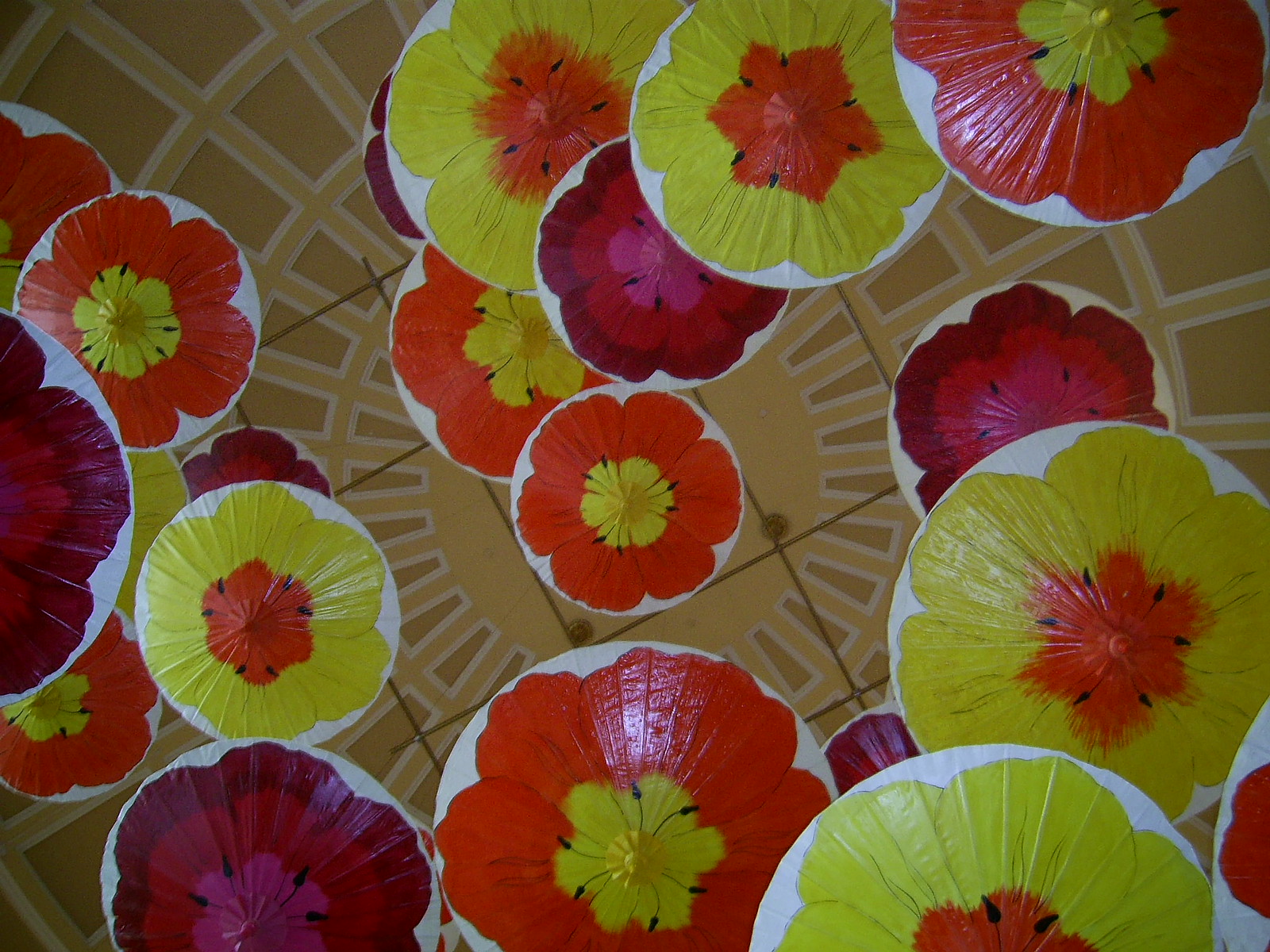The image appears to be a vibrant, artistic collage featuring numerous small, cut-out illustrations of flowers, each encircled by a thin white border that accentuates the petals. The flowers, presented in a variety of sizes, predominantly showcase hues of orange, yellow, and red, with intricate variations where some have yellow petals with red centers, others displaying red petals with yellow centers, and a few showcasing pink or lavender tones. Each flower consistently has six petals. These floral illustrations are haphazardly scattered across what resembles a concentric and geometrically patterned background. The backdrop itself features pale orange and dark orange rectangles, resembling elements seen in an extravagant architectural ceiling, possibly hinting at the ornate design of a museum or a historic building. The entire composition creates a striking juxtaposition of the organic beauty of flowers against a structured, almost architectural framework, enriching the visual appeal with detailed textures and vivid colors.